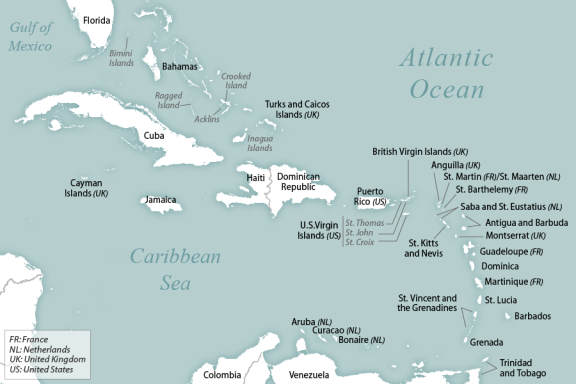This is a detailed map of the Caribbean region, highlighting several geographical elements and labeled locations. The map features a pale blue background for the ocean. The Atlantic Ocean is marked in blue text at the top right, while the Caribbean Sea is labeled in the bottom left. The Gulf of Mexico is identified in the top left corner.

At the very top left, we see the tip of Florida. Directly beneath Florida are the Bahamas, followed by the long landmass of Cuba. Under Cuba, there is Jamaica and the Cayman Islands (UK). To the right of these islands, the map shows Haiti and the Dominican Republic side by side. Continuing rightward, we see Puerto Rico (US), and further right, several islands including the British Virgin Islands (UK), Anguilla (UK), Saint Martin (France), Sint Maarten (Netherlands), Saint Barthélemy (France), Saba and Saint Eustatius (Netherlands), Antigua and Barbuda, Montserrat (UK), Guadeloupe (France), Dominica, Martinique (France), Saint Lucia, Barbados, Saint Vincent and the Grenadines, Grenada, and Trinidad and Tobago.

In the bottom part of the map, connected to the continent of South America, we find Colombia and Venezuela. North of these South American countries are the Dutch islands of Aruba, Curaçao, and Bonaire. Underneath Puerto Rico are the US Virgin Islands, labeled Saint Thomas, Saint John, and Saint Croix.

Near the top of the map, several smaller gray-labeled islands include the Bimini Islands, Ragged Island, Acklins, Inagua Island, and Crooked Island. The map also includes a legend at the bottom left, which defines FR as France, NL as Netherlands, UK as United Kingdom, and US as United States.